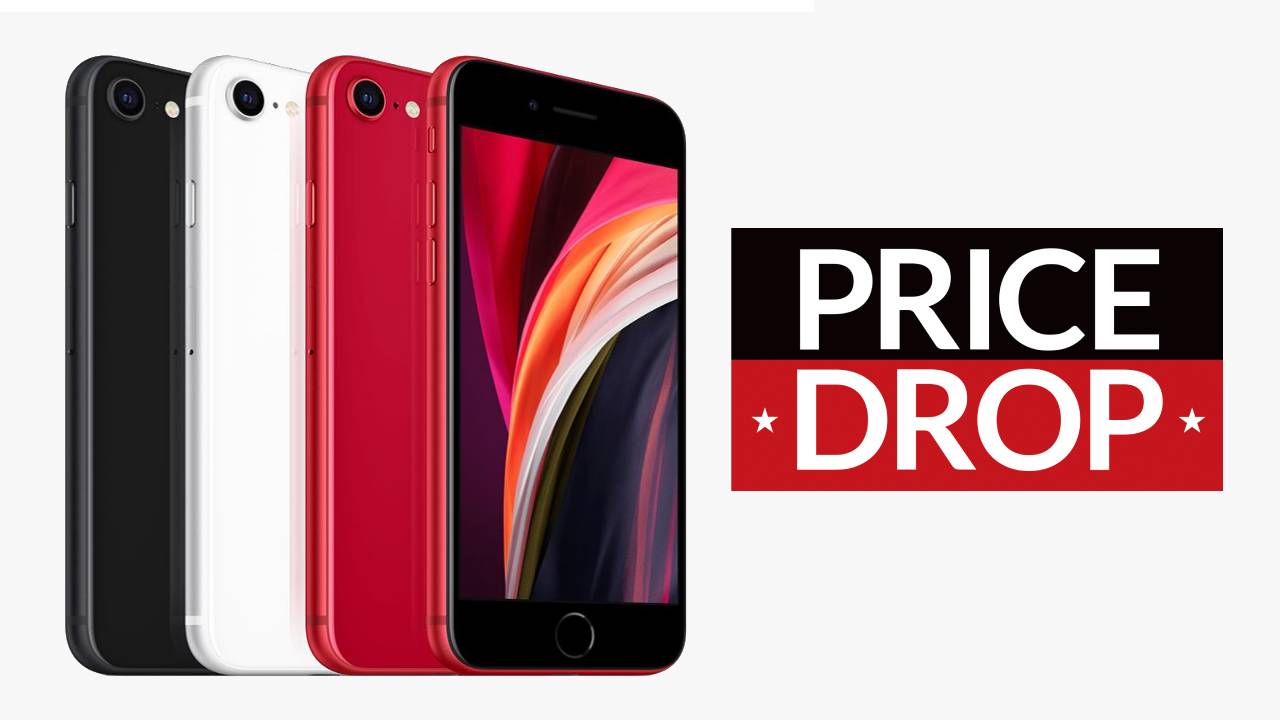The image features a white background with a dynamic arrangement of four smartphones on the left. The phones are staggered diagonally to showcase their cases. From left to right, the lineup includes a black smartphone, followed by white, red, and another red smartphone. Unlike the others, the red smartphone at the far right is turned around to display its vibrant screen, which features an eye-catching design of red, orange, white, and yellow swirls. On the right side of the image, there is a prominent rectangular banner. The top half of this rectangle is black, and it contains the word "PRICE" in bold white letters. The bottom half is red and features the word "DROP" also in bold white letters, flanked by white stars on either side. The overall image is wider than it is tall, balancing product display with promotional messaging.